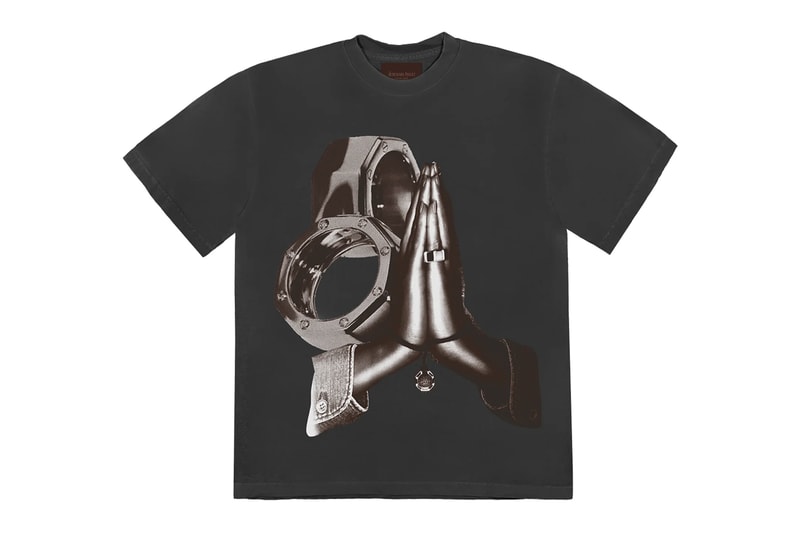This image features a black t-shirt, displayed against a plain white backdrop to emphasize its design. The t-shirt is laid flat, showcasing its crew neckline and the large, intricate graphic dominating the front. The graphic appears in various shades of silver, from dark to light, depicting a pair of delicate, praying women's hands. The left hand is adorned with a prominent ring on the pinky, while both wrists are wrapped with a black string featuring a small, circular metallic pendant. Additionally, the figure's sleeves suggest a denim shirt, visible through the detailed cuffs and buttons. Flanking the praying hands are two large, shiny octagonal objects, resembling oversized rings or bolts, adorned with tiny jewels at each corner. These metallic objects add a striking, industrial flair to the design, with one partially see-through, revealing elements of the shirt beneath.